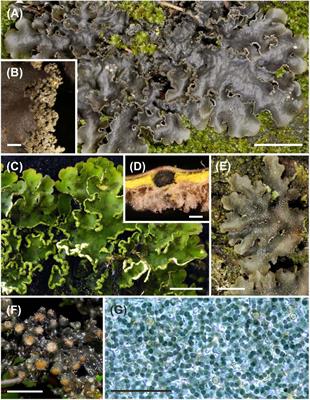This collection consists of several color images labeled A through G, each capturing distinct natural elements and objects. 

- **Image A**: Showcases a dark gray, leafy material resting atop vibrant green moss. This material resembles a lichen or a similar organism, suggesting a symbiotic relationship in a moist, forested environment.
- **Image B**: Features a brown item with irregular, jagged edges. The texture and shape hint at natural origins, possibly a piece of tree bark or a dried leaf.
- **Image C**: Displays a green, leafy plant characterized by dark green foliage with white borders. The plant might evoke a superficial resemblance to lettuce, but its distinct leaf pattern indicates a different species.
- **Image D**: Presents a yellowish-brown object of unknown origin. The object's texture and color are ambiguous, leaving room for speculation about its nature.
- **Image E**: Provides a close-up view of the dark grayish-green leafy material observed in Image A, enhancing the details of its texture and structure.
- **Image F**: Focuses on a collection of small black spheres, whose uniformity in shape suggests they might be seeds or spores.
- **Image G**: Appears to be a microscopic image revealing a mesmerizing swirling pattern composed of light blues, dark blues, and whites, evoking the beauty of abstract art or the intricacies of cellular structures.